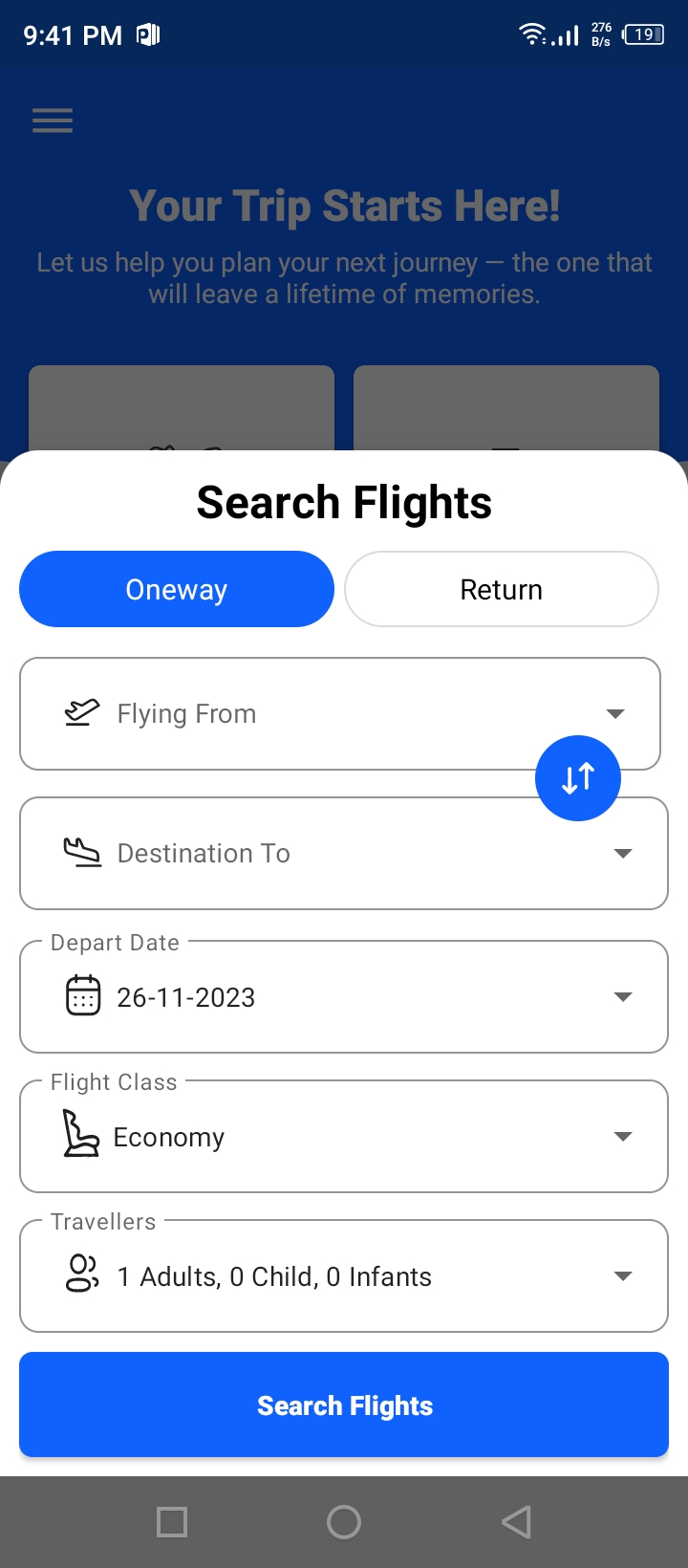The screenshot displays a mobile phone screen with a navy blue banner at the top, showing the time as 9:41 PM. To the left, a square icon contains the letter "P," while the right side features indicators for battery life (19%), Wi-Fi signal, and a status signal displaying "276 B/s."

Below the banner, arranged in three horizontal lines, is a center-aligned text area. In gray text, an exclamation invites the user with "Your trip starts here!" Directly underneath, an encouraging message reads, "Let us help you plan your next journey, one that will leave a lifetime of memories."

The primary content area includes two gray square tabs which are mostly obscured by a prominent white pop-up overlay. This overlay features a search form dedicated to finding flights. At the top, the text "Search flights" appears. Below are two selectable options: "One Way" on a blue background with white text, and "Return" on a white background with black text. 

Five drop-down menus provide the user with flight details: 

1. "Flying from,"
2. "Destination to."

These two are connected by a circle with an up and down arrow between them. The subsequent drop-down fields include:

3. "Depart date" set to "26-11-2023,"
4. "Flight class" as "Economy,"
5. "Travelers" indicating "1 adult, 0 children, 0 infants."

A clickable blue banner at the bottom of the pop-up reads "Search flights" in white text, positioned above a footer banner consisting of a square, a circle in the middle, and a right-facing triangle or arrow.